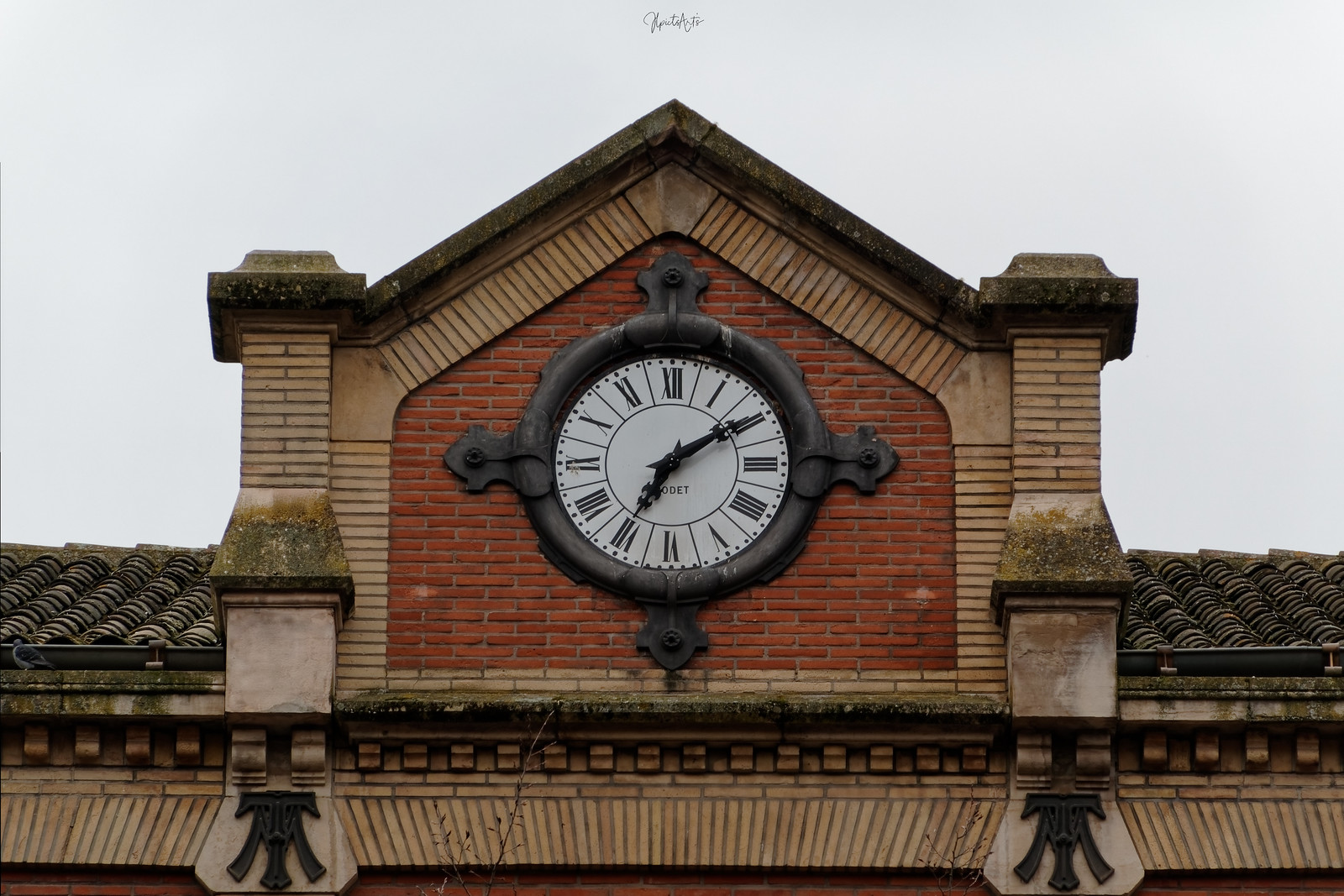The photograph captures an outdoor clock mounted at the peak of a historic building's roof. The sky in the background is pale and washed out, providing a neutral canvas, above which the photograph is signed in an unreadable, spidery script.

The roof, composed of weathered terracotta tiles, features a prominent triangular dormer-like structure. This structure is framed by stone and yellow brick columns on either side, with a stone slab forming the peak of the roof. The yellow brick subsequently forms an inner border, creating a house-like outline. The interior is filled with red brick, providing a stark contrast. 

The clock itself, large and round, appears to be made of cast iron or oil-rubbed bronze. It is mounted onto the red brick with four intricately designed three-lobed floral brackets positioned at the twelve, three, six, and nine o’clock positions. The clock face is white with black Roman numerals, and it has three hands indicating the hours, minutes, and seconds.

Below this structure, the lower part of the roof is adorned with detailed dental molding at the eaves. At the base of the two columns flanking the clock, there are decorative stone elements reminiscent of a tie knot, narrow at the top and broad at the bottom. Metal decorations, matching the brown hue of the clock, adorn the left and right sides of the structure, completing the intricate and historical aesthetic of this architectural feature.